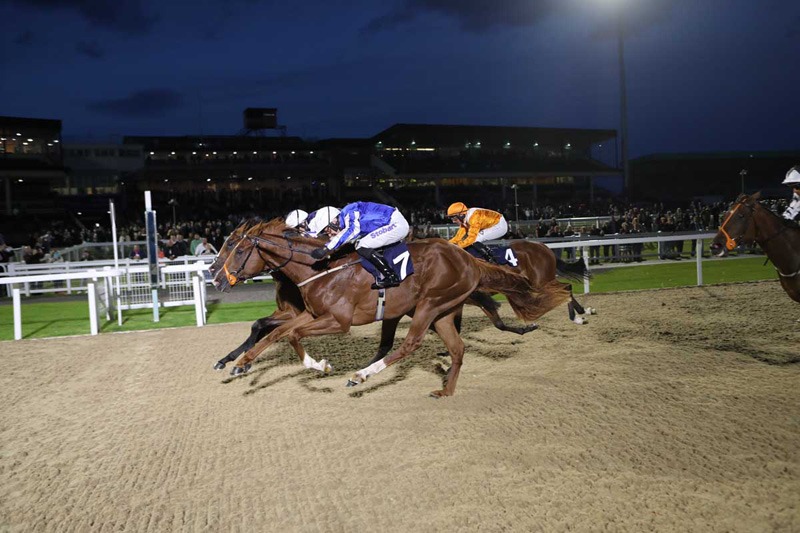The image is a color photograph taken from a nighttime horse race, captured as a video freeze-frame in landscape orientation. Central to the image are four brown horses in mid-stride, racing on a light-colored dirt track. The two leading horses appear to be in a dead heat; both are the same shade of brown. The horse on the far right, partially cut off, is slightly darker. The foremost horse, wearing number seven, is ridden by a jockey in a blue top with white pants, while the jockey on the horse directly behind is in a white top. A third horse, numbered four, is slightly behind them, managed by a jockey in a shiny golden-yellow jersey. The backdrop features a white barrier, a green grass field, and the stands filled with spectators. The dark blue sky overhead, tinged with purplish hues, indicates it's nighttime, with bright floodlights illuminating the scene. The stands in the distance reveal multiple story levels and a glowing light source in the top right corner.